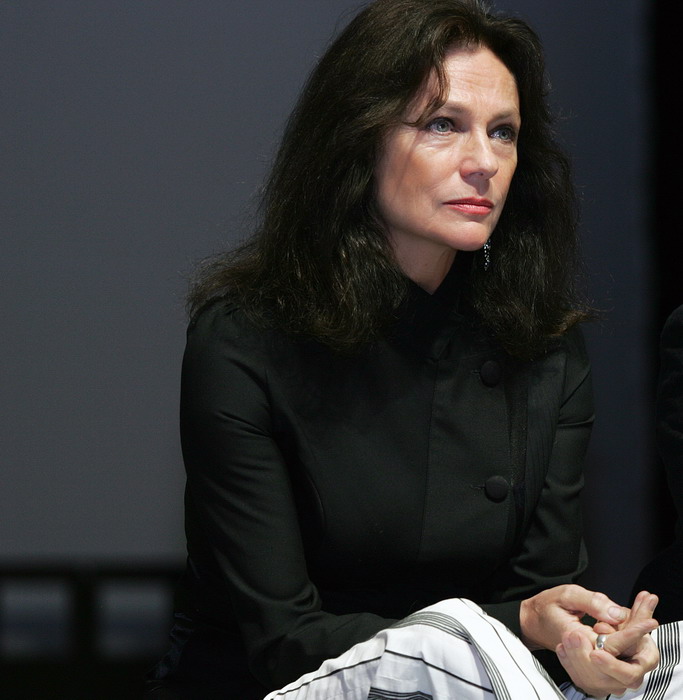In an image characterized by a subtly blurred, charcoal-grey background, the central focus is an older to middle-aged woman who commands attention with her striking presence. Her long, jet-black hair frames a fair complexion, accentuated by the vivid red of her lipstick. Dangling earrings add a touch of elegance, complementing her composed expression as she gazes directly ahead. She dons a stylish, long-sleeved black top paired with white pants adorned with black stripes, creating a sophisticated monochromatic ensemble. Her hands are clasped together, and a silver ring gleams discreetly on one of her fingers, contributing to her poised and polished appearance.